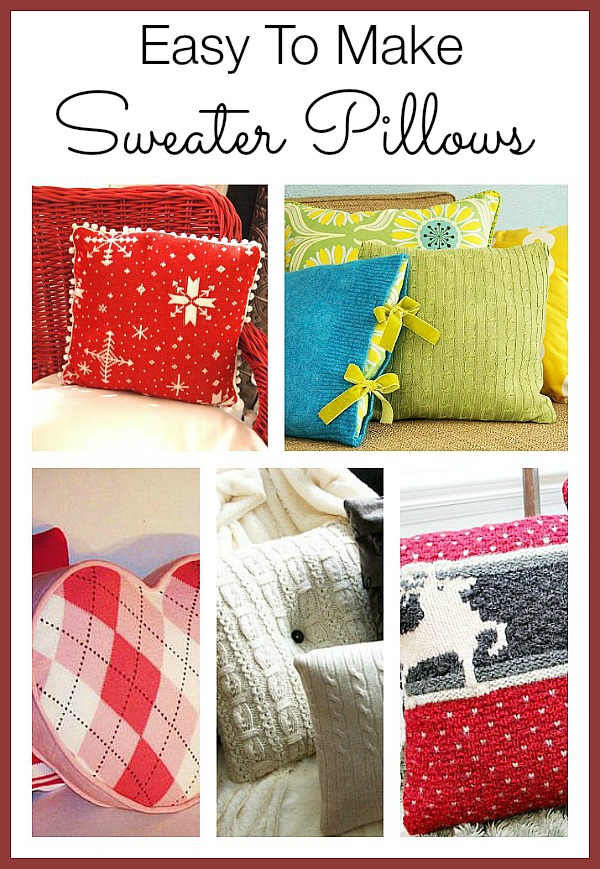Title: Easy to Make Sweater Pillows

Description: The image is a detailed guide on crafting sweater pillows, featuring a collage of five distinct designs. The top left pillow is red with festive white snowflake or star patterns, evoking a cozy, holiday spirit. Adjacent to it on the top right, three pillows draw attention with their unique colors and designs: a solid blue pillow resembling a sweater, a lime green pillow, and a mixed-patterned green and blue pillow with a yellow floral motif in the background. The bottom row showcases a variety of creative shapes and patterns. On the left, a heart-shaped pink pillow adorned with a checkerboard pattern in shades of red, pink, and white, perfect for Valentine's Day. The center pillow is a classic white cable-knit design with a central black button, mimicking a real sweater's texture. Lastly, the right pillow features a distinctive striped design with red and pink borders and a gray center, displaying a white reindeer - reminiscent of an 'ugly sweater' pattern. The entire composition is framed by a red border, enhancing the festive and cozy theme aptly described by the guide’s title.